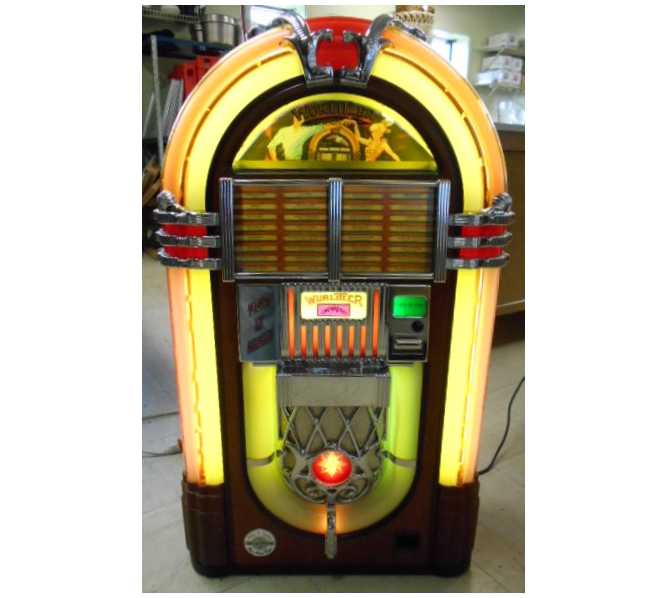The image features an old-style jukebox prominently positioned in the center of a light-colored tile floor. This vintage jukebox stands about counter-height, around 4 to 5 feet tall, and is adorned with a mix of wood inlays and wood base. Vibrant yellow fluorescent tubes curve around the entire jukebox, complemented by red, silver, and orange accents. The upper section houses a playlist display for song selection, below which is a coin slot and speaker. Above the playlists, encased in glass, is a painted image of a couple dancing in front of another jukebox, enhancing its nostalgic charm. In the backdrop, despite being out of focus, shelves filled with various items like paper towels and cooking utensils suggest a setting resembling a storage room or possibly the back area of a store or restaurant.